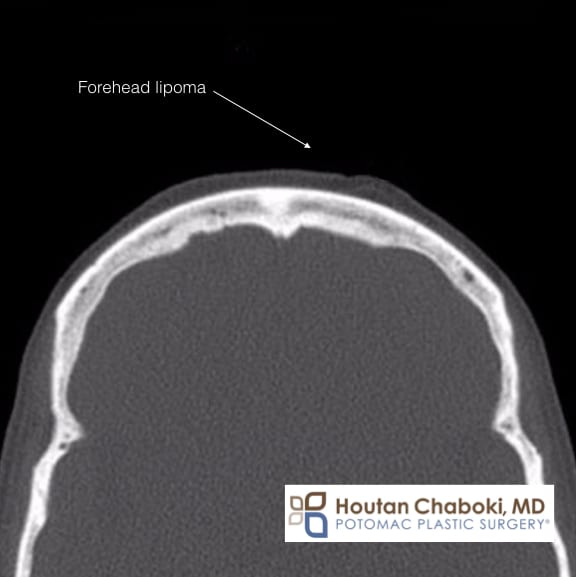The image is a rectangular, black-background x-ray of a cross-section of someone's head, primarily showing the upper skull region. The top of the head is rounded, with a noticeable bump labeled "forehead lipoma," accompanied by an arrow pointing to it. Surrounding the bump are white lines delineating the skull structure, creating a half-moon shape from the bottom left to the bottom right of the image. The anatomical features, such as the bone outline, are clearly visible, while the interior organs are indistinct and blurry, adding to the diagnostic focus on bone and skin.

In the bottom right corner, there is a rectangular white box containing the name "Hutan Chibaki, MD," identified as a Potomac plastic surgeon. To the left of this text is a distinctive design associated with his practice. Additionally, there are colorful circles in each corner of the image: a blue circle in the bottom right, a gray circle in the top right, a light gray circle in the bottom left, and a dark gray circle in the top left. These elements, combined with the label and detailed imaging, suggest that the picture is both an advertisement and a diagnostic reference for treatments provided by Dr. Chibaki's plastic surgery practice.